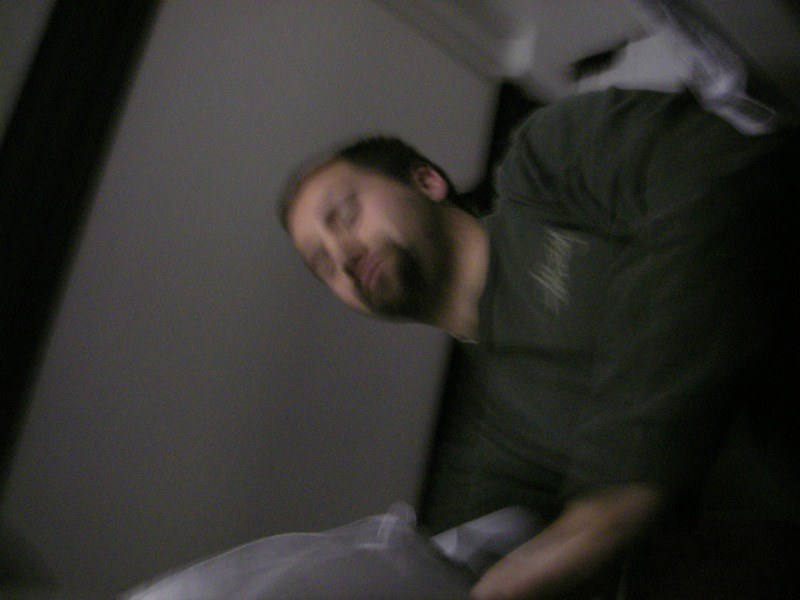This grainy, blurry image features a man sitting down, rotated 90 degrees anti-clockwise. The man is wearing a green long-sleeved T-shirt or sweatshirt. His eyes are closed, and his head is gently tilted backward, giving him a peaceful or slightly smiling expression. He has short, dark hair along with a short mustache and beard. In the background, a white wall is visible, with a black or brown edge of an object running along it. In front of the man is a white piece of cloth or fabric, also blurry and hard to identify. On the top left area of his chest, his sweatshirt has writing in a white or light color, featuring a street art style that is not fully legible.